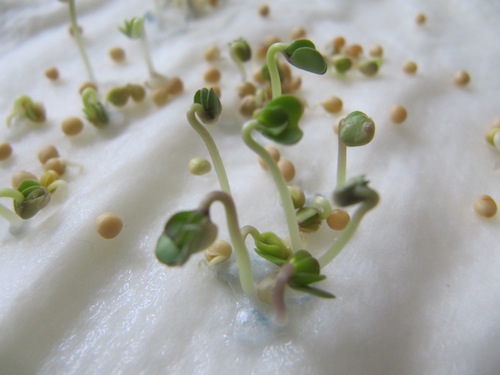The photograph captures a close-up view of several sprouting plants emerging through a moisture-retaining, man-made surface that appears to be made from a textured styrofoam or plastic material. The sprouting plants, which resemble bean plants, feature light green stems and small green pods. Scattered across the surface are numerous round spheres that look like peas, some of which are brown and partially split open, revealing white nubs. The sprouts are about an inch tall with two small green leaves at the top, indicating they are in the early stages of growth. In the background, a few shorter sprouts can be seen, suggesting a varying rate of germination among the seeds.